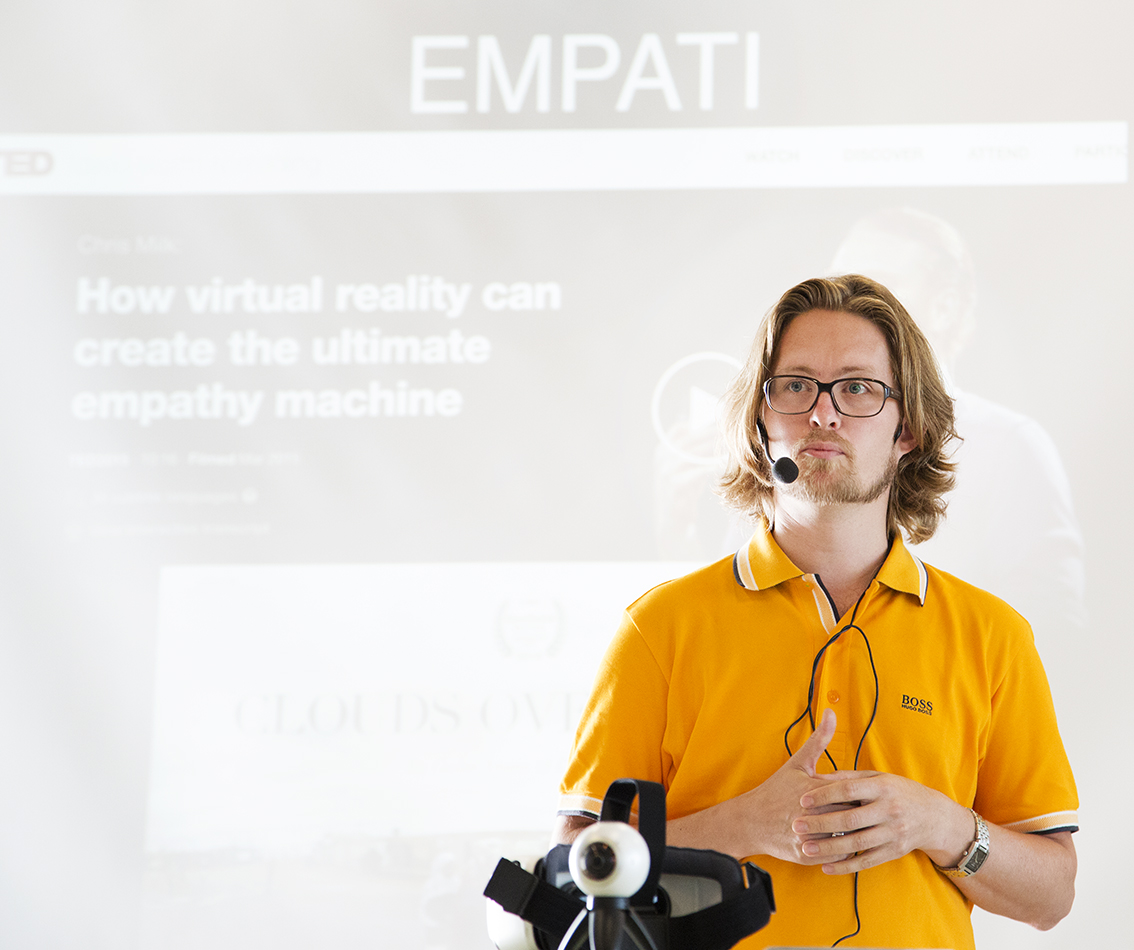In the foreground of the image, there's a man, likely presenting at an event, standing in front of a projection screen. The man is wearing a short-sleeved, collared yellow shirt emblazoned with the logo "Boss." He has shoulder-length blonde hair and a bit of brown facial hair. A wire from his microphone runs behind his neck and down his chest. He wears glasses, a wristwatch, and holds his hands together near chest level. In front of him is an intriguing device resembling an eyeball on a pole with some virtual reality glasses positioned behind it. 

The background features a large projector screen displaying a slide. The slide has a grayish and whitish color scheme, with the title "Empati" at the top in white font. Below this heading, a subtitle reads, "How Virtual Reality Can Create the Ultimate Empathy Machine." The detailed surroundings of the man have been cropped out, emphasizing the presentation's focus on virtual reality technology.